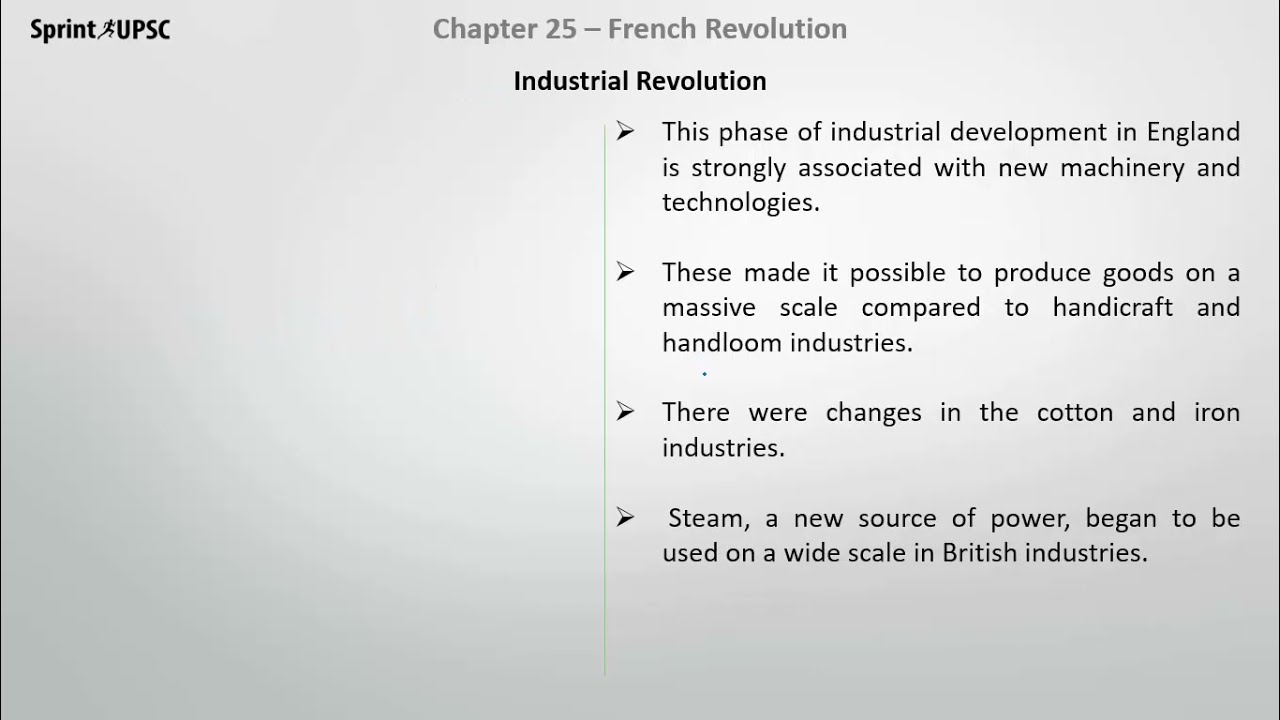The image is a grayscale screen capture, possibly from an online lesson or a digital text, resembling an informational card or PowerPoint slide. The upper left corner features the word “sprint” in black text, accompanied by an icon of a sprinter or runner, and the acronym “UPSC”, all set against a gray background. Centrally positioned at the top in medium gray text is the title "Chapter 25 - French Revolution," and directly underneath in black text is the subheading "Industrial Revolution."

The left side of the image is mostly blank except for the aforementioned elements, contrasted by a vertical divider separating it from the right side where content is displayed. This right side consists of three bullet points marked with small arrows, and four detailed paragraphs. 

1. The first paragraph states, "This phase of industrial development in England is strongly associated with new machinery and technologies."
2. The second paragraph explains, "These made it possible to produce goods on a massive scale compared to handicraft and handloom industries."
3. The third paragraph notes, "There were changes in the cotton and iron industries."
4. The fourth paragraph highlights, "Steam, a new source of power, began to be used on a wide scale in British industries."

This card provides an overview of the Industrial Revolution in the context of the French Revolution chapter, illustrating key changes in Britain’s industrial landscape.